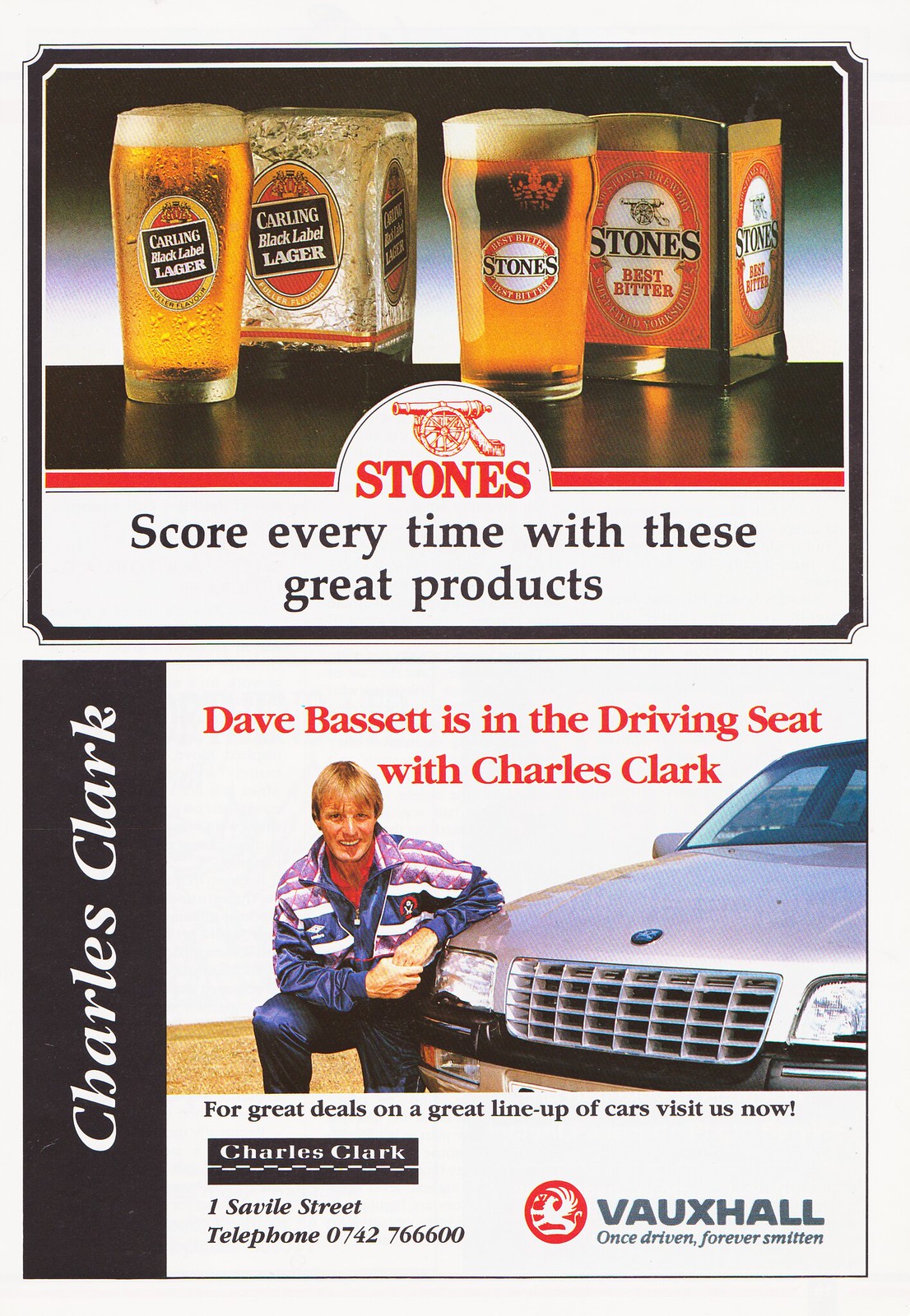The image is divided into two sections. The top section features two glasses of beer filled to the brim, glowing golden under the light. The glass on the left is labeled "Carling Black Label" in white text, while the glass on the right proudly displays the "Stones" logo, which consists of black lettering on a white background, encircled by orange banners stating "Best Bitter" at both the top and bottom. Each glass is accompanied by a corresponding box; the Stones box is particularly striking with its gold color and red or orange horizontal label. The beer in the glass has about an inch of white, foamy head, and everything is set on a dark surface.

The bottom section of the image contrasts this with a different advertisement: a person seated next to a silver car. The ad text highlights Dave Bassett being "in the driving seat with Charles Clark," indicating a car promotion. This distinct segmentation of the image creates a dual-focus advertisement, one celebrating beer brands and the other marketing a car.